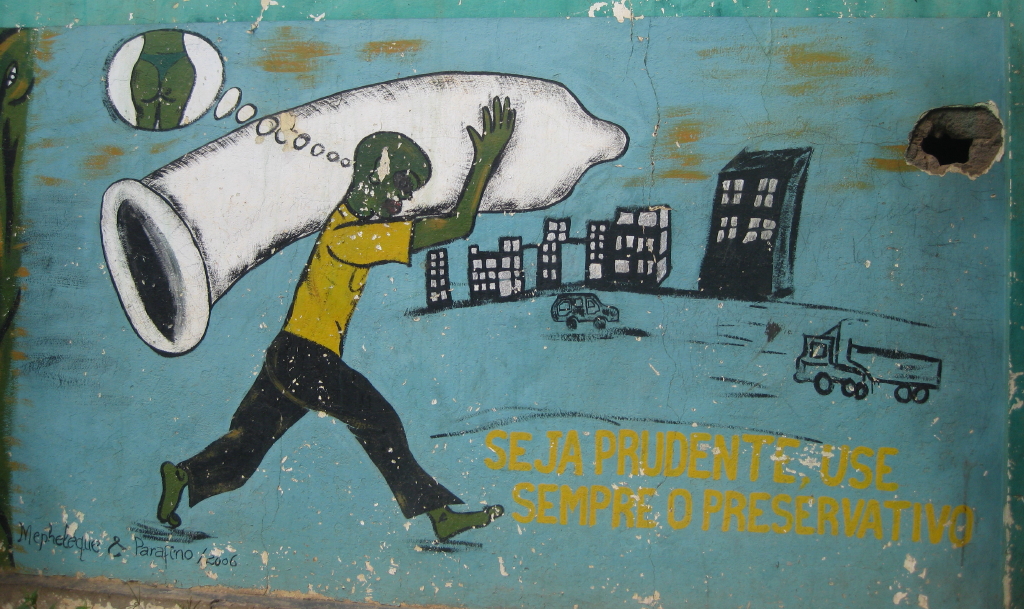The artwork, created by Meheke Parafino in 2006, depicts a crudely drawn, barefoot green man walking through a cityscape with black-and-white buildings, a car, and a truck in the background. The man, wearing a yellow shirt and black pants, carries an oversized, unrolled condom slung over his left shoulder. Emerging from his head is a thought bubble containing the image of a woman's buttocks clad in a thong. The scene includes a Spanish caption in yellow letters at the bottom right corner, which reads, "Seja prudente, use siempre o preservativo," emphasizing the importance of prudent and consistent use of condoms.